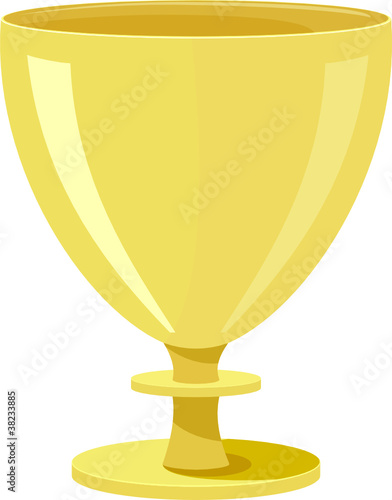This stock photo features an illustrated golden chalice or goblet, centrally positioned against an all-white background. The image, rendered in simple, lineless colors that evoke the style of a children's cartoon, includes subtle highlights and shadows. Light is depicted through white streaks along the sides and a yellow streak that accents the cup's gold coloring. The goblet has a round base, a thick stem, and a slightly smaller circle above the base. Across the image is a watermark reading "Adobe stock," with the identifier "number 38233885" appearing along the left side, indicating its position within Adobe's extensive image collection. The faded gray text across the illustration ensures the image remains protected until purchased.